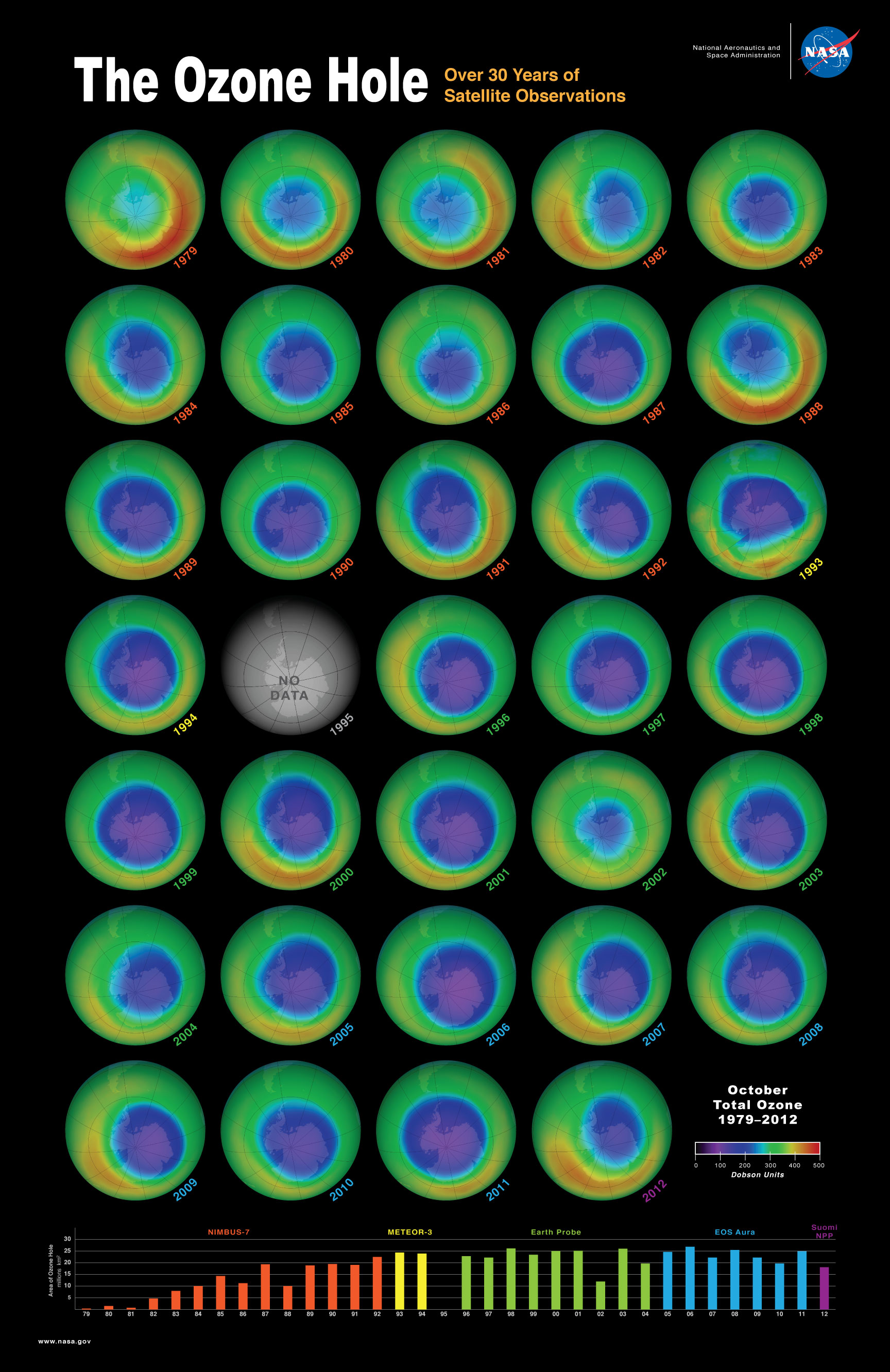This poster is a detailed informational display focused on "The Ozone Hole: Over 30 Years of Satellite Observations". Set against a black background, the upper right-hand corner features the NASA logo and the word "NASA," accompanied by the title "The Ozone Hole" in white font. The main body of the poster consists of a grid of approximately 40 circular images arranged in five horizontal circles per row over about eight rows. Each circle represents Earth, with a lighter green background and varying central blue areas depicting the size and shape of the ozone hole over different years, denoted by orange year labels that are admittedly hard to read. Notably, one circle in the fourth row from the left is marked as "no data," indicating missing information for that period.

At the bottom of the poster is a horizontal bar graph that visually complements the circular images above. This graph starts with red on the left and transitions through yellow and green to end with blue, likely representing changes in data related to the ozone hole across the observed years from 1979 to 2012. Though the specific details of what the bar graph measures are too small to read, it visually reinforces the progression and magnitude of changes in the ozone layer over the given time period.